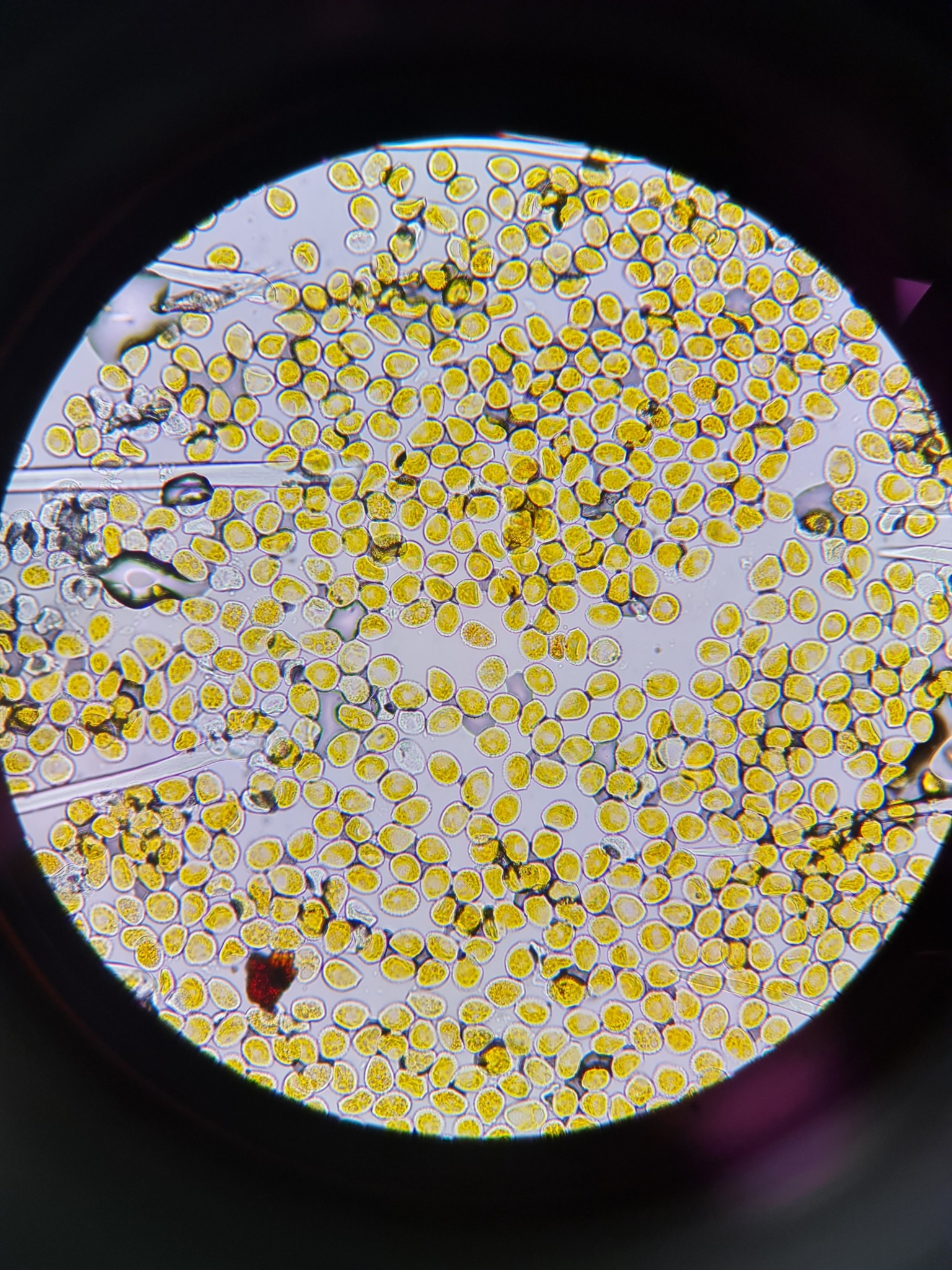This image, captured through an optical light microscope, displays a highly detailed view of microscopic cells or bacteria. The overall composition is a square rectangle with a primarily black background that frames a circular field of view. Within this circular area, the background is a clear-ish gray, and it is densely populated with approximately 200 small, yellow, and somewhat spherical cells that are not perfectly shaped. Each yellow cell contains darker granules and is outlined by a purple ring. 

Several long, clear needle-like structures intersect the microscopic field: three emanate from the left and one crosses the top of the sphere, while two more intrude from the right but only extend about a third of the way. Additionally, there is a distinctive reddish-purple blob-like structure situated in the bottom left part of the circle, which is likely some form of debris. The image, with no text present, spans the majority of the width, giving a professional and detailed visual representation of the microscopic world.